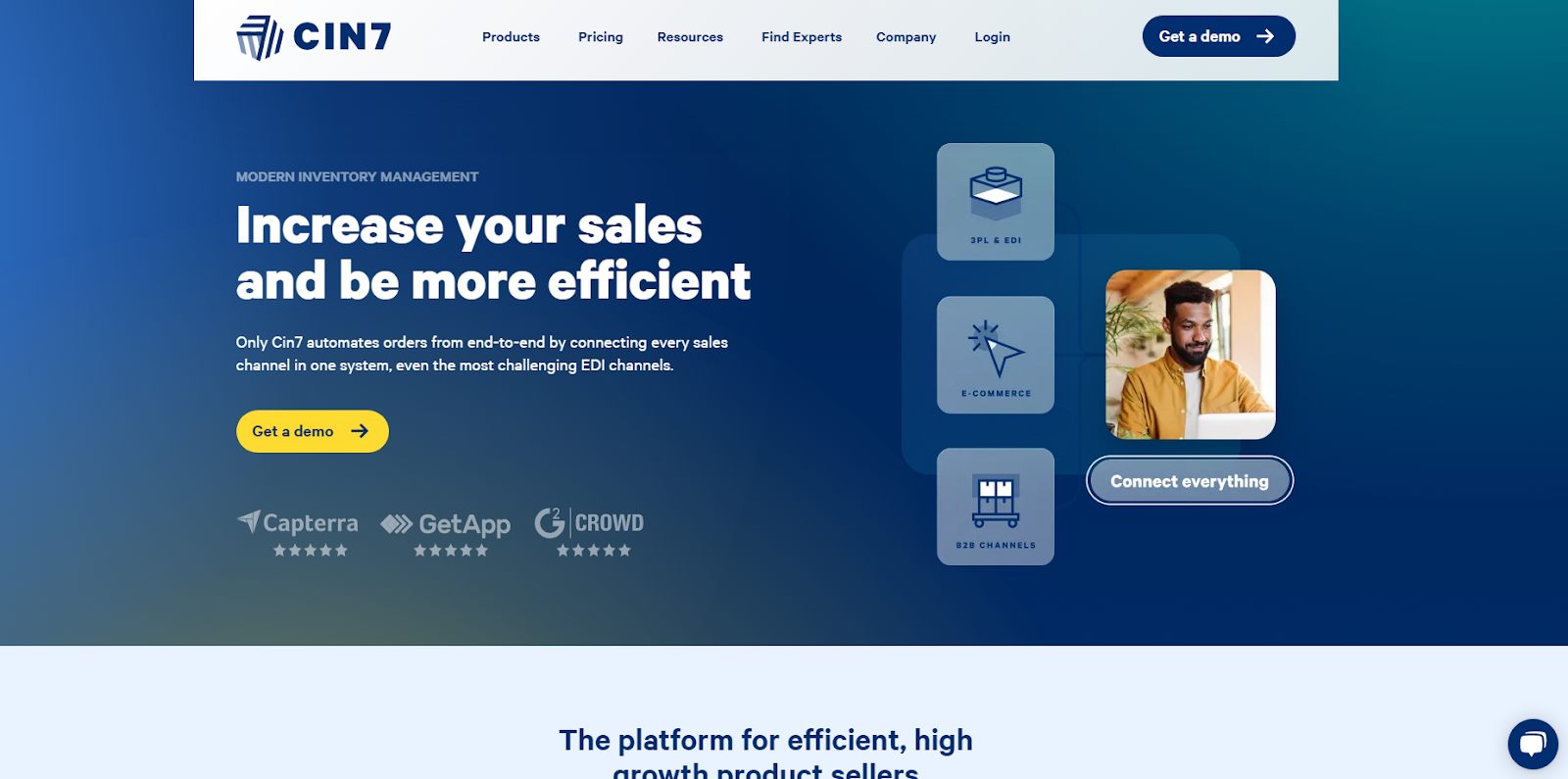The image prominently displays the logo "CIN7" at the top, with a geometric shape adjacent to it, all set within a whitish box. To the right of this logo, a navigation bar presents the options: "Products," "Pricing," "Resources," "Find Experts," "Company," and "Login." Below this, a blue button with white text invites users to "Get a Demo."

Central to the image, bold white text reads: "Increase your sales and be more efficient," just below the tagline: "Modern Inventory Management." The text further explains that "Only CIN7 automates orders from end to end by connecting every sales channel in one system, even the most challenging EDI channels." Additionally, a yellow button again prompts users to "Get a Demo."

Underneath, the image showcases credibility with icons depicting five-star ratings from CapTera, GetApp, and G2 Crowd. Adjacent to this section, on the right side, are three vertically aligned boxes featuring various icons, each representing different functionalities or features. Below these boxes is a photograph of a person dressed in an orange jacket, accompanied by a button labeled "Connect Everything."

The bottom part of the image is a light blue section that reads in blue text: "The platform for efficient high growth product sellers." In the bottom right corner, there's a blue bubble containing white speech bubbles, enhancing the image's emphasis on communication and connectivity.